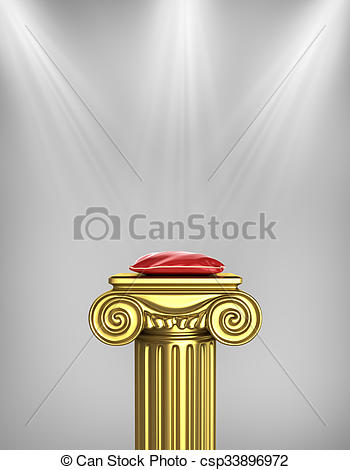This is a detailed stock photo featuring a cartoon image that resembles an envelope on its side, rendered as a vertical rectangle in gray. The corners of the image have lines converging towards the center, mimicking the appearance of an envelope. Central to the image is a darker, outline drawing of a camera set horizontally, with the text "CAN STOCK" next to it, forming a watermark. Below this central watermark, there is an intricate gold podium adorned with scrolling decorations along its front. Atop the golden podium sits a small, square, dark red pillow, likely made of silk or velvet, featuring white trim around its edges. This trim is thin and adds a delicate accent to the cushion. The pillow and podium are set against a backdrop that gives the impression of a white photographic backdrop. Beneath the main image, there is a line of text that reads "Copyright Can Stock Photo" followed by CSP33896972. The image also includes subtle elements like faint lines that draw attention towards the watermark and three lights at the top illuminating the pillow.